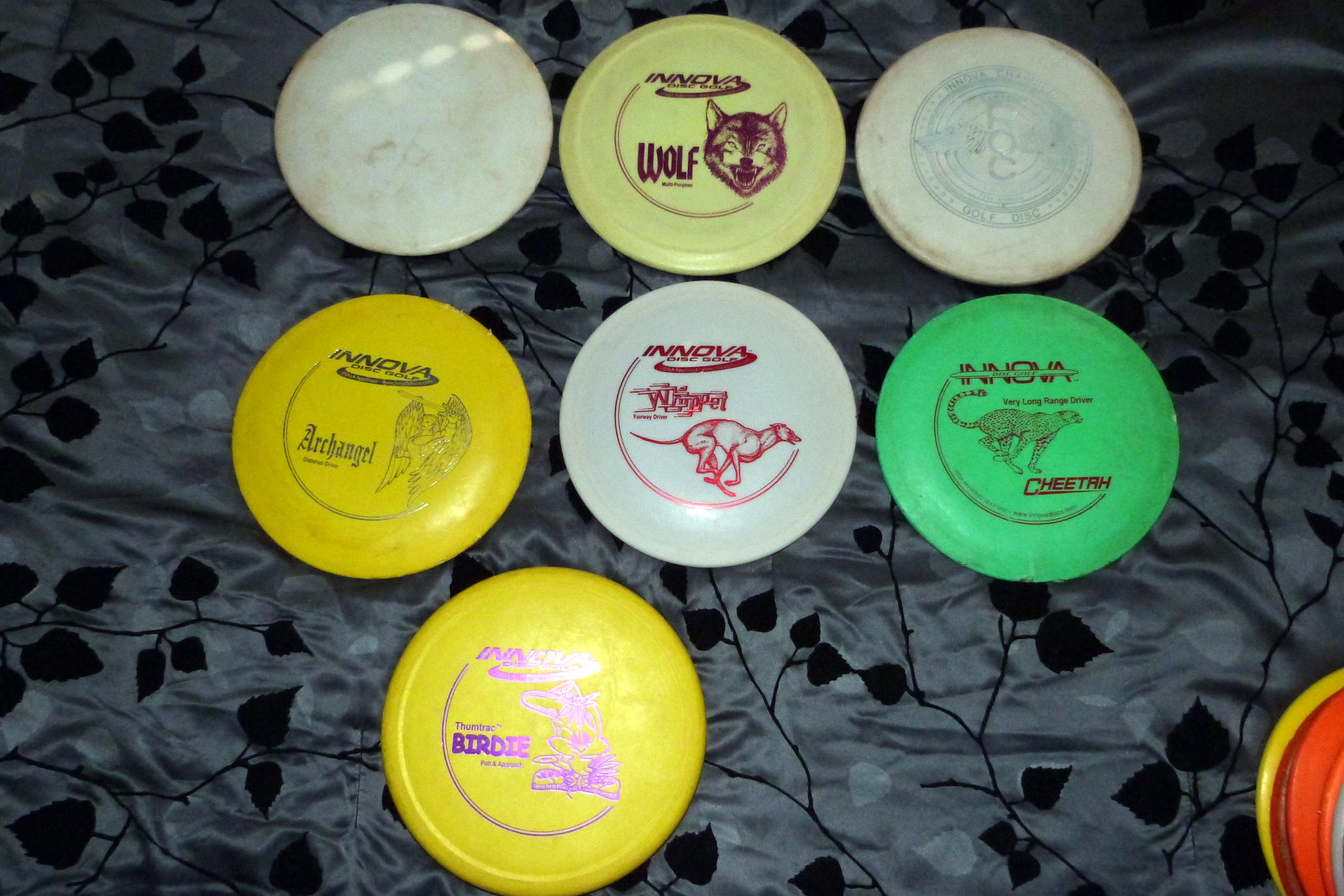This image portrays a collection of disc golf frisbees meticulously arranged on a silky, silver-gray bedspread adorned with a black leaf pattern. Centered in the photograph are seven prominent frisbees, organized in three rows: three at the top, three in the middle, and one at the bottom. Additionally, a stack of frisbees with their edges visible lies in the bottom right corner.

The frisbees are primarily of the Innova brand and each bears distinct markings and designs:
- **Top Row**: 
  - The leftmost frisbee is plain white and visibly dirty with mud or dirt marks.
  - The center frisbee is light yellow with maroon text that reads "Innova Disc Golf" and "Wolf," accompanied by an image of a wolf.
  - The rightmost frisbee is white with a faded, circular bluish design, also marked with "Innova Disc Golf."

- **Middle Row**: 
  - The first frisbee on the left is bright yellow featuring an "Innova Disc Golf" logo and an illustration of an angel wielding a sword, labeled "Archangel."
  - The middle frisbee is white with "Innova Disc Golf" text in red and an image of a dog, identified as a "Whippet."
  - The rightmost frisbee is green with the label "Cheetah" beneath an image of a cheetah.

- **Bottom Row**:
  - The lone frisbee here is bright yellow, labeled "Thumb Track Birdie," adorned with a cartoon bird in purple.

In the lower right corner, additional frisbees can be seen with their edges peeking into the frame, displaying a mix of colors including yellow, red, orange, and gray.

Overall, the image captures a diverse array of frisbees featuring different colors and intricate designs, all laid out neatly on a dark, leafy-patterned bedspread.